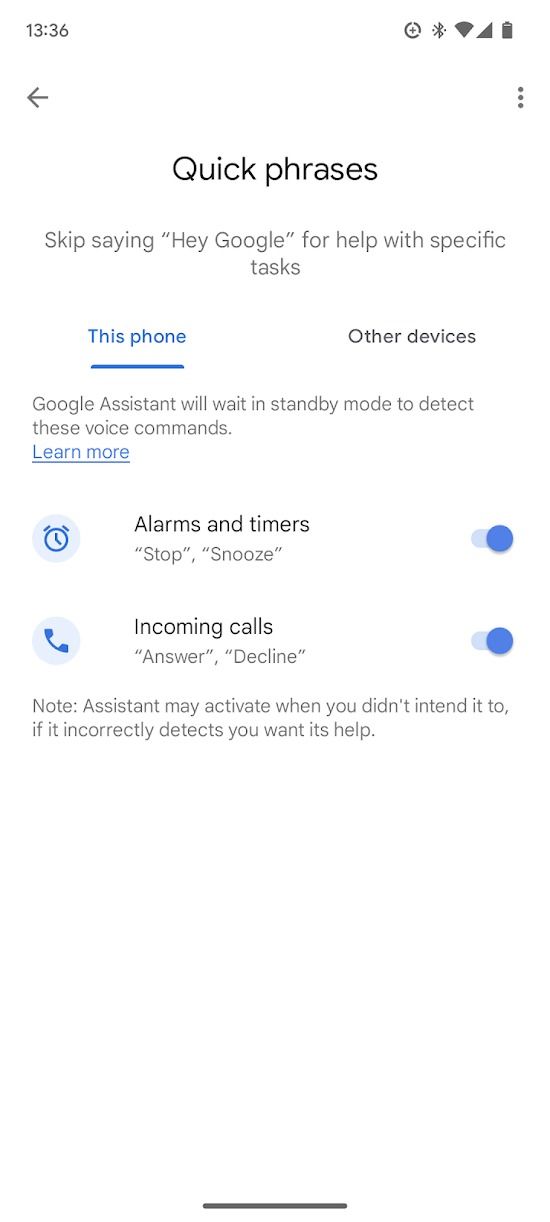A detailed descriptive caption for the provided cell phone screenshot would be:

"The screenshot captures the display of a smartphone at 1:36 PM. The device is connected to Bluetooth and Wi-Fi, has full cell phone signal bars, and an almost fully charged battery indicated in the upper right corner. Just below these icons, a gray left-pointing arrow represents the back button, and on the opposite side, three vertical dots signify a drop-down menu. The screen title, 'Quick Phrases,' is displayed prominently in black text. Directly beneath it, a message in gray text reads, 'Skip saying "Hey Google" for help with specific tasks.' The screen further divides into two categories: 'This Phone,' labeled in blue, and 'Other Devices,' not highlighted. Below these tabs, another gray message states, 'Google Assistant will wait in standby mode to detect these voice commands,' with a blue 'Learn More' hyperlink for additional information. The subsequent section lists features activated with blue icons and toggle switches to the right. The first feature, represented by a blue alarm clock icon, reads, 'Alarms and timers: stop, snooze,' with its toggle switch turned on. The second feature, marked by a blue phone icon, states, 'Incoming calls: answer, decline,' also with an active blue toggle switch. At the bottom of the screen, a cautionary note advises, 'Assistant may activate when you didn’t intend to, if it incorrectly detects you want its help.'"